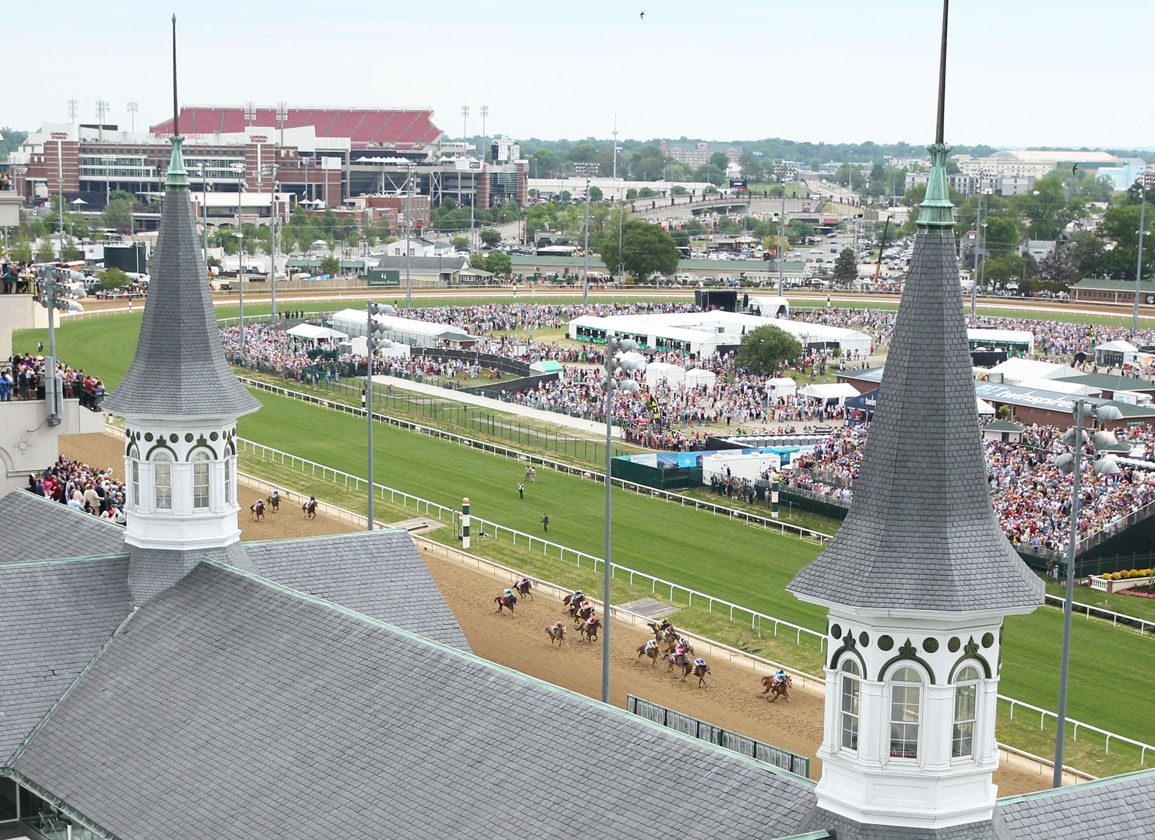The photograph captures a lively horse race scene with a large, ornate building in the foreground featuring a gray roof adorned with two prominent spires. The race track is bustling with action as several horses race along the brown dirt track, which is bordered by a white railing. Inside the track, there's a meticulously maintained green infield encircled by another railing. The infield is densely packed with spectators, suggesting a high-profile event, possibly like the Kentucky Derby. The stands are full, indicating a significant turnout. Additional structures, possibly stables or tents, are visible within the infield, hinting at amenities for horses and participants. Beyond the immediate race venue, the background reveals other buildings and trees, contributing to a populous and bustling atmosphere.